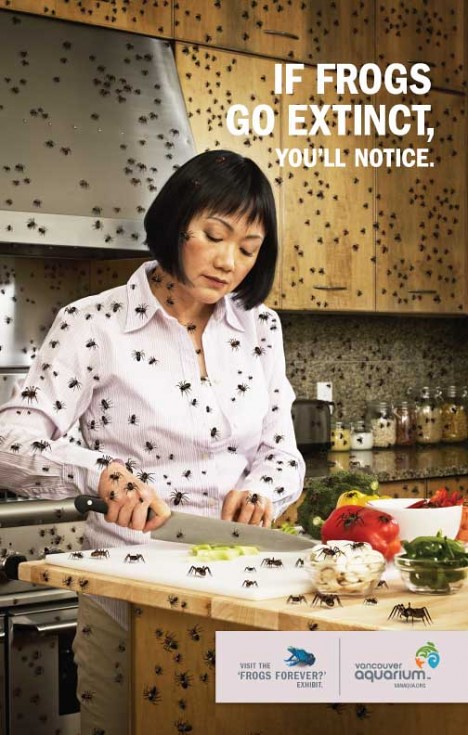This vivid and unsettling poster features an Asian woman with black hair in her early 50s, standing in her kitchen and focusing intently on chopping an array of vegetables, including peppers, mushrooms, lettuce, and broccoli, which are laid out on a cutting board on a wooden counter. The kitchen is furnished with everyday items such as an oven and a toaster visible in the background.

However, the scene takes a disturbing turn with swarms of insects—including crickets, ants, and spiders—crawling all over the woman and the kitchen. These unsettling creatures are on her face, shirt, hands, and pants, as well as scattered across the kitchen counter and walls. The poster's message is starkly displayed in white text at the top: "If frogs go extinct you'll notice." Below, additional text encourages viewers to "Visit the Frogs Forever exhibit at Vancouver Aquarium," accompanied by a small logo featuring a blue frog.